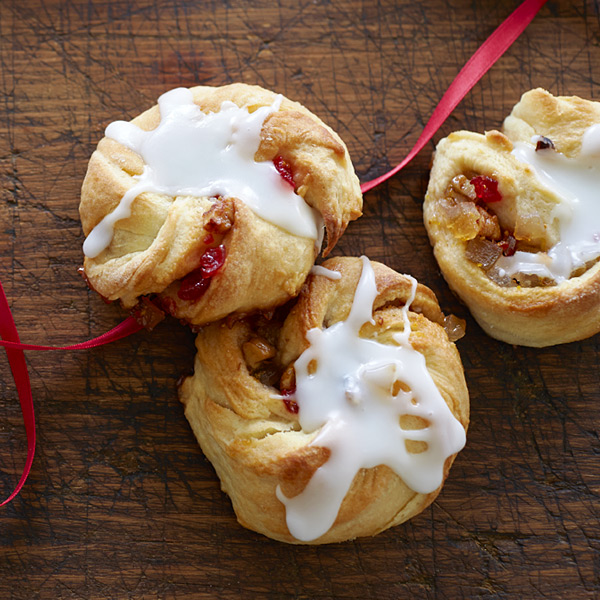This indoor photograph captures a close-up view of three small, round pastries arranged on a heavily worn wooden table. The medium brown table, which is covered with numerous dark gouges and cuts, acts as a rustic backdrop for the pastries. Each pastry is made from a crescent-type dough, baked to a light brown with golden edges. They are filled with a mixture of red berry filling and nuts. A white glaze that has hardened as it cooled is drizzled over the tops of the pastries. Some of the red berry filling and nuts are visible through the cracks of the dough, adding a touch of color and texture. A thin red ribbon stretches diagonally from the lower left to the upper right corner, threading beneath the pastries and adding a festive accent to the scene.